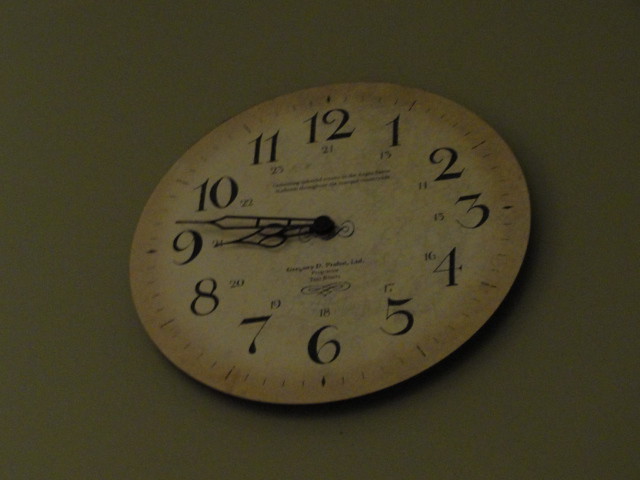This image showcases a vintage-style clock face with an antiqued tan background, evoking an age-old charm. The clock features traditional Arabic numerals from 1 to 12 displayed clearly around the dial. In addition to the standard time markings, the clock also includes military time notations positioned beneath and slightly to the left of each corresponding hour numeral. For example, beneath the 12 is the military figure "24", beneath the 1 is "13", and so forth, allowing for quick reference to the 24-hour format. Notably absent is a second hand, leaving only the hour and minute hands. The time displayed on the clock shows the hour hand pointing at 9 and the minute hand nearing 47 minutes past the hour, indicating the current time as either 9:47 PM/military time 21:47, or 9:47 AM.